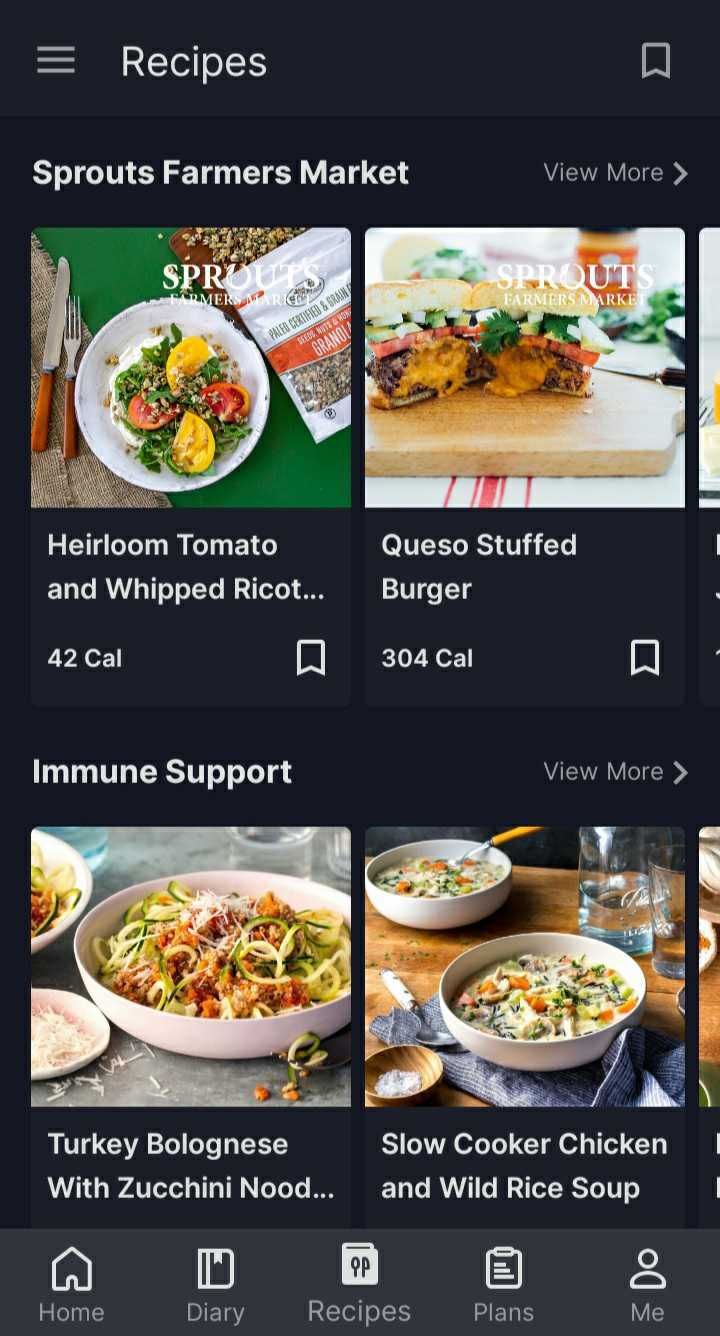A vibrant and delicious spread featuring heirloom tomatoes, both red and yellow, artfully displayed on a plate. Accompanying the tomatoes is a whipped ricotta and queso stuffed cheeseburger, an enticing dish with only 304 calories. The scene also includes a healthy option of turkey bologna served with zucchini noodles, perfect for immune support. In addition, there's a bowl of slow-cooked chicken and wild rice soup, making for a hearty and comforting meal. The background is a striking black, with white text adding a modern touch. This beautifully crafted image captures the essence of fresh ingredients and mouth-watering recipes, inviting you to explore more culinary delights from your home diary and meal plans.